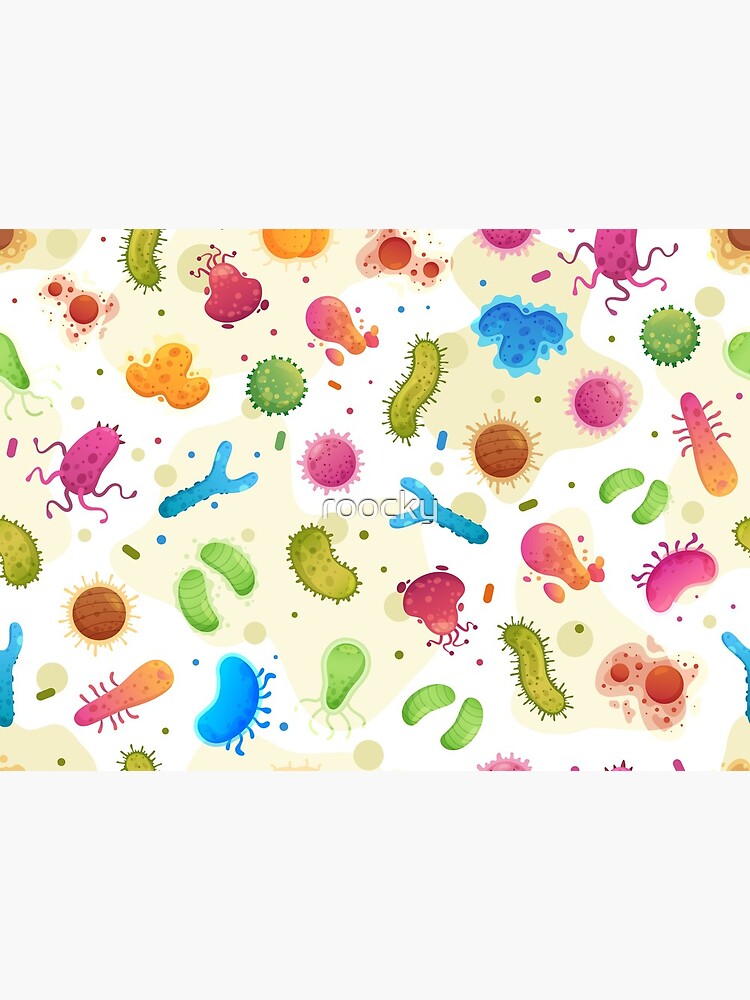The image depicts what appears to be wallpaper or wrapping paper, characterized by a white background teeming with colorful, animated bugs or paramecium-like shapes. There are various vividly colored germs, ranging in hues from green, pink, orange, blue, red, and brown. Each bug has distinctive features: green bugs with multiple legs, little lime-colored worm-like shapes, and orange ones dotted with specks. Some bugs are round with spikes, often in pink, while others resemble wishbones in blue or simple round red objects. A unique green bug with longer legs stands out among them. Scattered throughout are tiny colored specks adding to the vibrant display. Prominently in the center, a watermark spells "R-O-O-C-K-Y," adding a distinct focal point amidst the colorful array. The image is bright and clear, providing a lively and engaging visual experience.